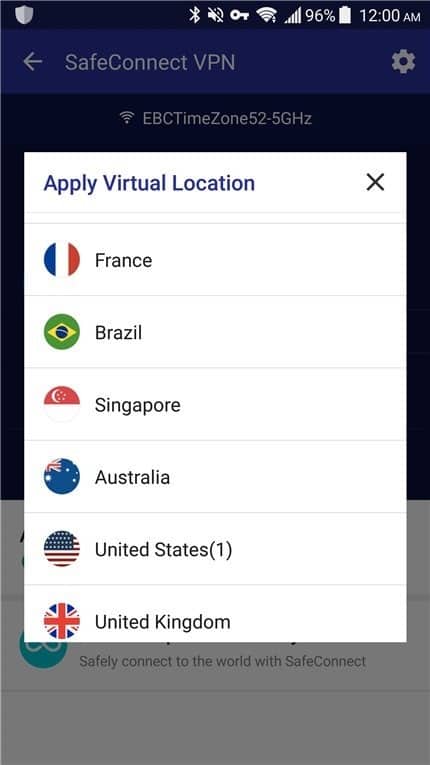Screenshot captured from a mobile phone display. At the top of the image, there is a thin black status bar. On the left side of this bar, a gray shield icon is visible, followed by icons indicating Bluetooth status, mute, a key, Wi-Fi strength, cellular signal, and a battery level at 96%. The time displayed is 12 AM.

Below the status bar, a dark blue header with gray text contains a back arrow, the words "Safe Connect VPN," and a gear icon. Against a darker blue background, the text shows Wi-Fi signal strength, the designation "EBC time zone 52-5 HG," and a lowercase 'z'.

A white pop-up window is prominently displayed, with the text "Apply Virtual Location" in black, along with a black 'X' on the right for closing the window. Below this pop-up, there are six circular icons representing different national flags: France, Brazil, Singapore, Australia, the United States (with a small '1' beside it), and the United Kingdom. The flags are in their respective colors, with the United Kingdom, France, Australia, and the United States having red, white, and blue; Brazil displaying green, yellow, blue, and white; and Singapore showing red and white.

The background beneath the pop-up is a lighter blue with readable text stating, "Safely connect to the world with Safe Connect."